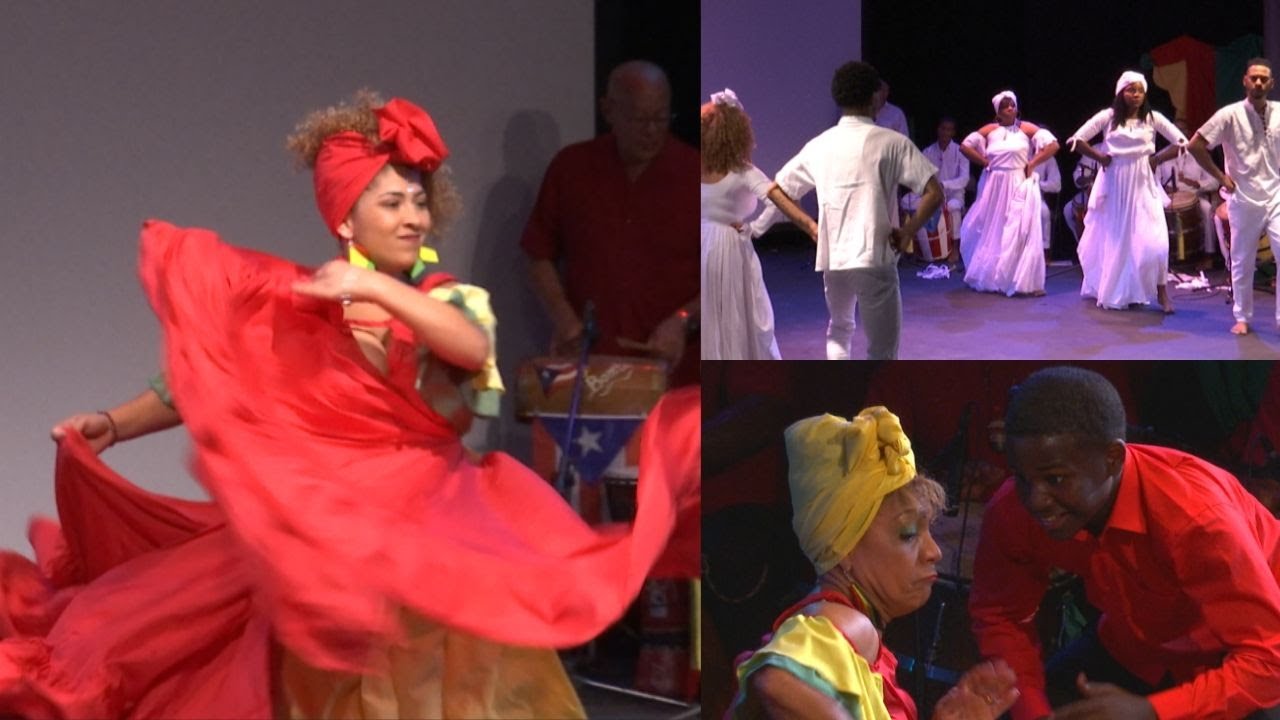This rectangular collage, approximately five to six inches wide and three inches high, is divided into three distinct parts, showcasing photographs taken indoors. The left side of the image features a larger photo of a stage production with a woman of light brown skin, wearing a yellow and red dress, dancing. She has curly light brown hair pulled up and adorned with a red turban-like head covering. The woman is captured mid-dance, holding and twirling her skirts. Behind her, a man with bald light brown skin, dressed in a short-sleeve red shirt, stands with some flagged object in front of him.

On the right half, the top photo shows a group of performers of African descent, clad in white outfits—white dresses and short-sleeve shirts—dancing with their hands on their hips, while a person in white plays drums in the background.

The bottom right image displays a conversation between a younger boy of African descent, wearing a long-sleeve red collared shirt, and a slightly older woman with light brown skin. The woman wears her hair up in a yellow scarf and sports a red, yellow, and green blouse. Together, these pictures capture dynamic and vivid moments of a culturally rich stage performance.